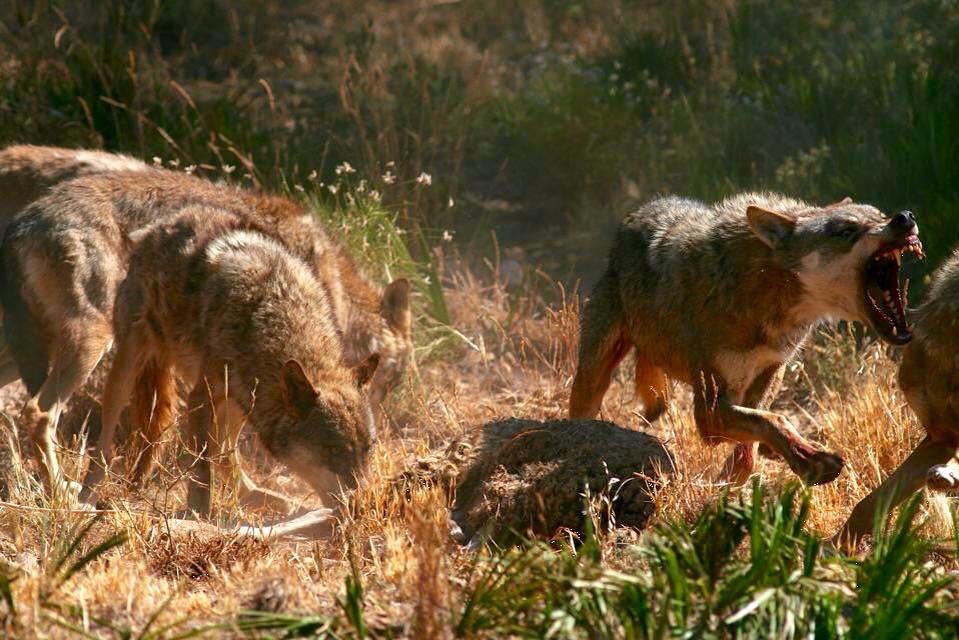In this image, we see a dynamic and intense scene set in a flat, grassy field with both green and brown hues. At the center of the image, a group of animals—likely hyenas or jackals—are engaged in a feeding frenzy on a dead animal. The animals have a vicious appearance, with some showing signs of blood on their fur. On the right, one of the creatures stands with a forward paw, mouth open, baring its teeth, casting a shadow that suggests the sun is not directly overhead. To the left, others are rooting around in the ground with their snouts. The backdrop reveals a small stream or river with a grassy embankment, adding to the natural setting. The scene is illuminated by daylight, yet partially shaded due to surrounding vegetation, indicating it's taken outdoors in the middle of the day. The colors in the image span different shades of brown, tan, green, black, red, and orange, adding to the vividness and rawness of this moment captured in nature.